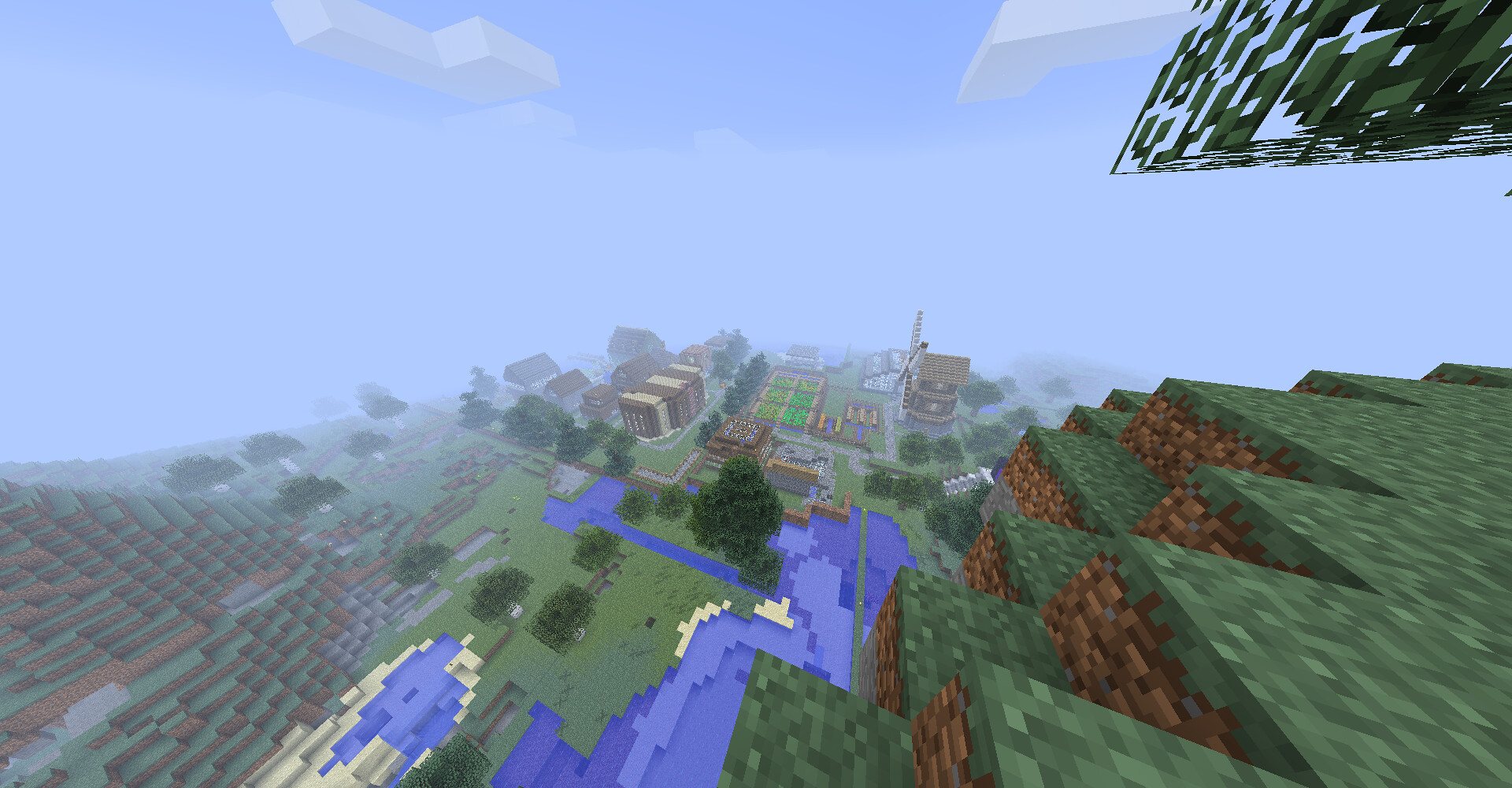This aerial screenshot from the game Minecraft showcases a vibrant and detailed vista. The scene captures the edge of a mountain or cliff with terraced, green and brown land formations stepping downward towards a valley. Dominating the middle of the image is a sprawling village featuring cultivated fields and two to three-story buildings. Noteworthy is a large windmill with visible blades and an angled roof nearby, adding a charming, rustic element to the village.

A clear blue sky occupies the upper half of the image, punctuated by blocky white clouds. A portion of a tree, with distinct cube-like leaves, is visible in the upper right corner, adding natural detail to the scene. A river or stream winds through the landscape, flanked by various hills and trees, contributing to the picturesque quality of this Minecraft landscape. Despite some pixelation, the scene is richly detailed, with a mix of residential and agricultural elements that give it a lively, bustling atmosphere.